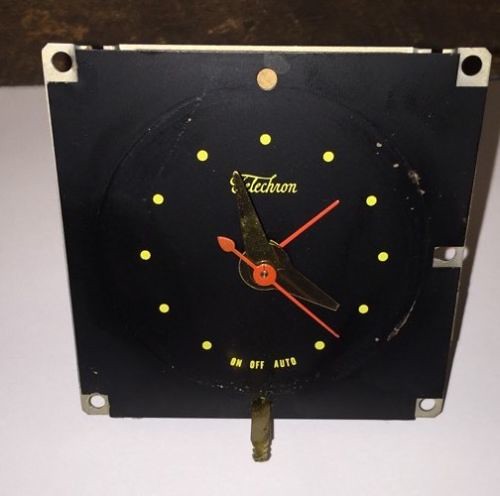The image showcases a unique black clock face devoid of traditional numerical markers. Instead, each hour is denoted by a small, distinct yellow dot. Prominently displayed are sleek black clock hands, partially obscuring the cursive brand name, possibly reading "Teletron" or a similar name. Accompanying the black hands are two vibrant red ones. At the bottom of the clock face, yellow inscriptions spell out "on," "off," and "auto." Each corner of the clock features circular metal cutouts, framed by a metallic structure. The base of the clock exhibits a bronze-like metallic section, adding a touch of elegance. The clock is placed on a pristine white table, set against a textured dark brown wall backdrop, enhancing the overall contrast and visual appeal of the scene.